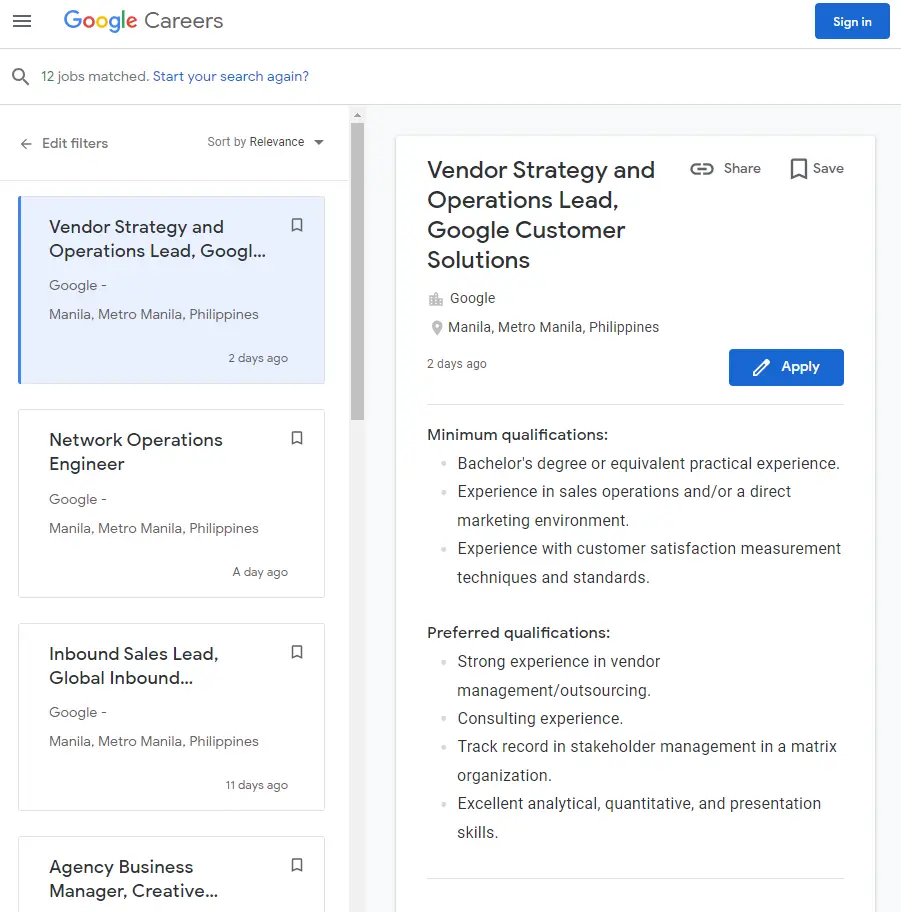The image displays a detailed view of a Google Careers page. In the upper left-hand corner, the vibrant Google logo stands out with its letters in distinct colors: a blue "G," red "o," yellow "o," blue "g," green "l," and a red "e," followed by the word "Careers" in gray. The top right-hand corner features a "Sign In" option for users.

On the left sidebar, there is an "Edit Filters" link, with a text above it stating "12 jobs match." Below, a blue link invites users to "Start your search again" if they’d like a fresh search.

Focusing on the job listings, the top job listing is highlighted in a blue square and reads "Vendor Strategy and Operations Lead" at Google, located in Manila, Metro Manila, Philippines. Following this, in white squares, are the listings for a "Network Operations Engineer" and an "Inbound Sales Lead, Global Inbound," both based in Google Manila, Metro Manila, Philippines. The next partial listing is for an "Agency Business Manager, Creative."

On the right-hand side of the page, a detailed job description for the "Vendor Strategy and Operations Lead" at Google Customer Solutions in Manila, Metro Manila, Philippines is provided. The position requires a minimum of a bachelor's degree or equivalent practical experience, along with relevant experience in sales operations, direct marketing environments, and customer satisfaction measurement techniques and standards. Preferred qualifications include strong experience in vendor management outsourcing, consulting, and a proven track record in stakeholder management within a matrix organization. Additionally, excellent analytical, quantitative, and presentation skills are highlighted.

Within this section, a blue rectangle provides a clickable "Apply" button, inviting potential candidates to submit their applications.